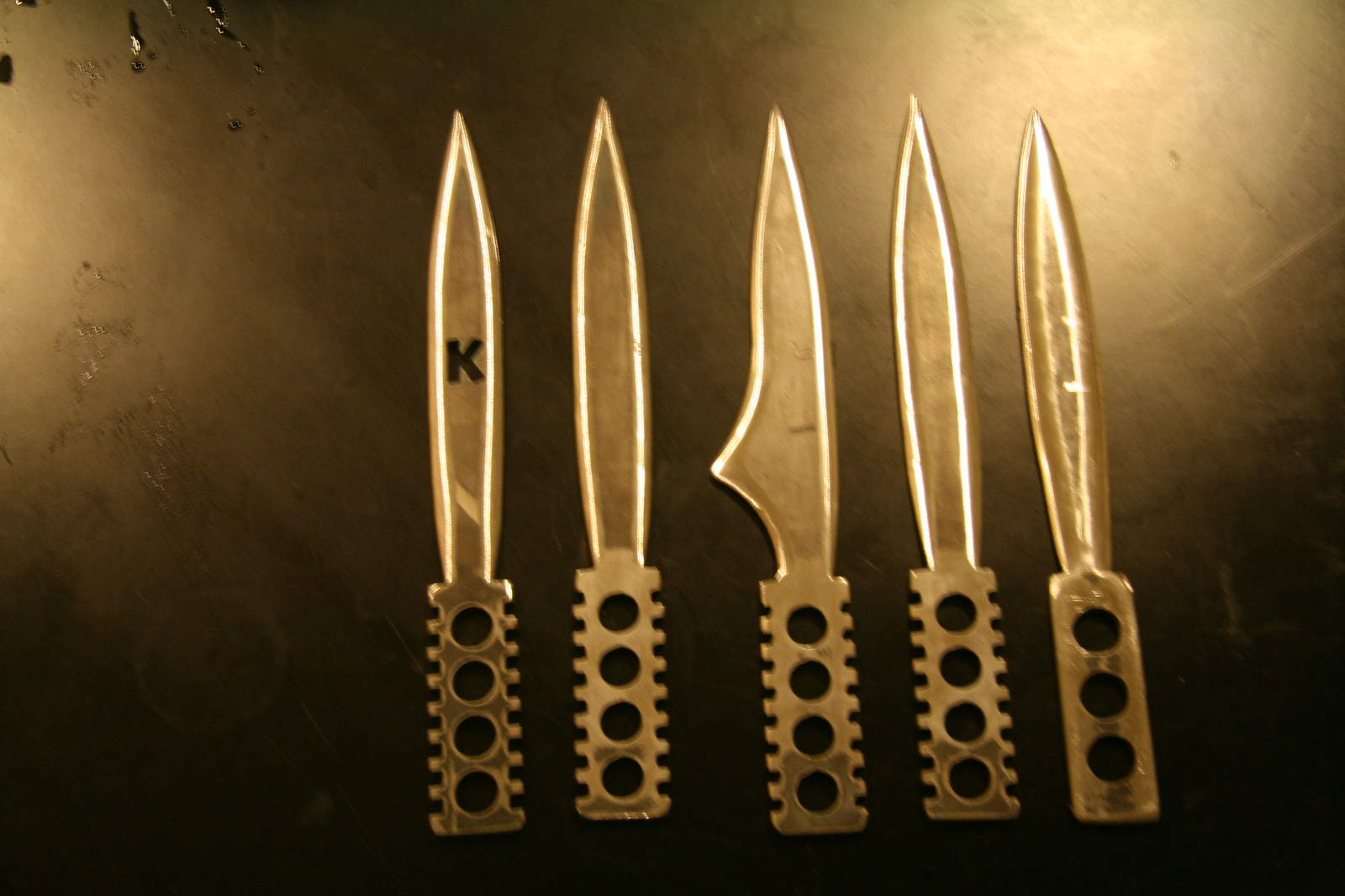This image features five brass-colored knife blades displayed in a row against a polished, burnished brass or goldish-brown surface. All the blades lack wooden handles, revealing simple metal handles with a distinctive hole pattern. The first four blades from the left have four evenly spaced holes and exhibit a corrugated edge, with small, squared-off ridges or teeth running down the sides of the handles. The rightmost blade, differing from the others, features only three holes and lacks the corrugated edges, presenting straight, smooth sides instead. The knife blades themselves are slender and pointed, though they do not appear to be sharpened to a cutting edge. Notably, the leftmost blade is marked with a black letter "K." The second blade is similar in shape to the first, while the third blade includes a unique triangular protrusion near the handle. The fourth blade is narrow, and the fifth blade is slightly wider at the base where it would be inserted into a holder. The entire set is highlighted with a subtle glow against the background, enhancing the intricate details of the metal.